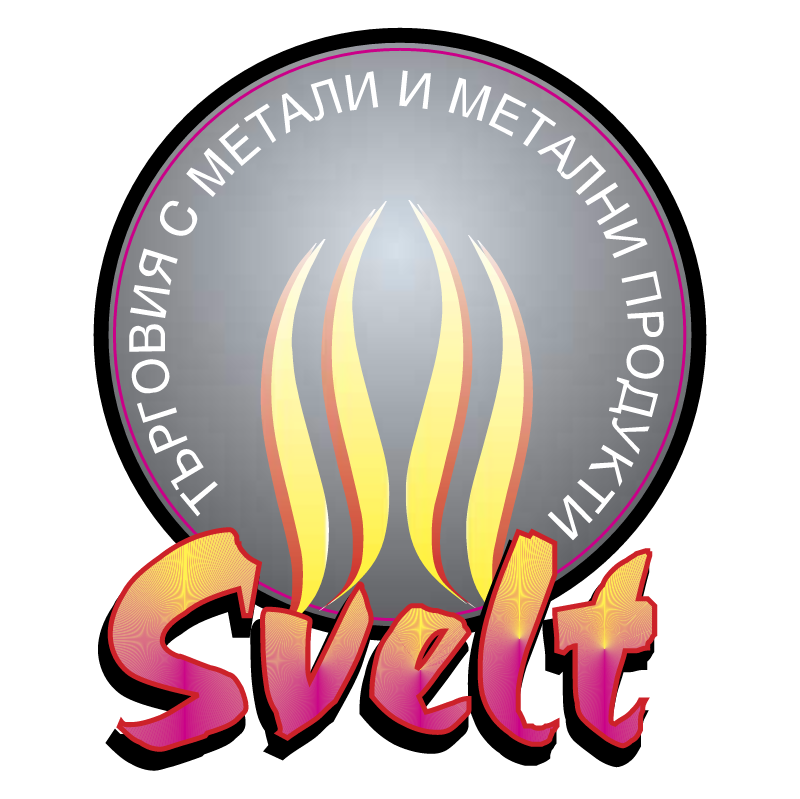The image features a prominently large circle bordered in black, with a thinner light purple border just inside. Along this purple border, arched white letters form an inscription, featuring characters such as 'T,' 'B,' 'P,' a backward 'N,' a backward 'R,' and 'C,' among others, spanning from the lower left to the lower right side of the arch. Within the black circle, the central area is gray, with notable yellow and orange flame shapes rising from the bottom towards the center; these flames exhibit a gradient, with orange on the outer edges and yellow internally. Below the circle, large block letters spell out "SVELT," with the lower part of these letters in a purplish-pink hue and the upper part in yellow. The contrasting colors and intricate design elements, including the foreign letters and symbolic flames, suggest that the image might be an advertisement or a logo in a different language.